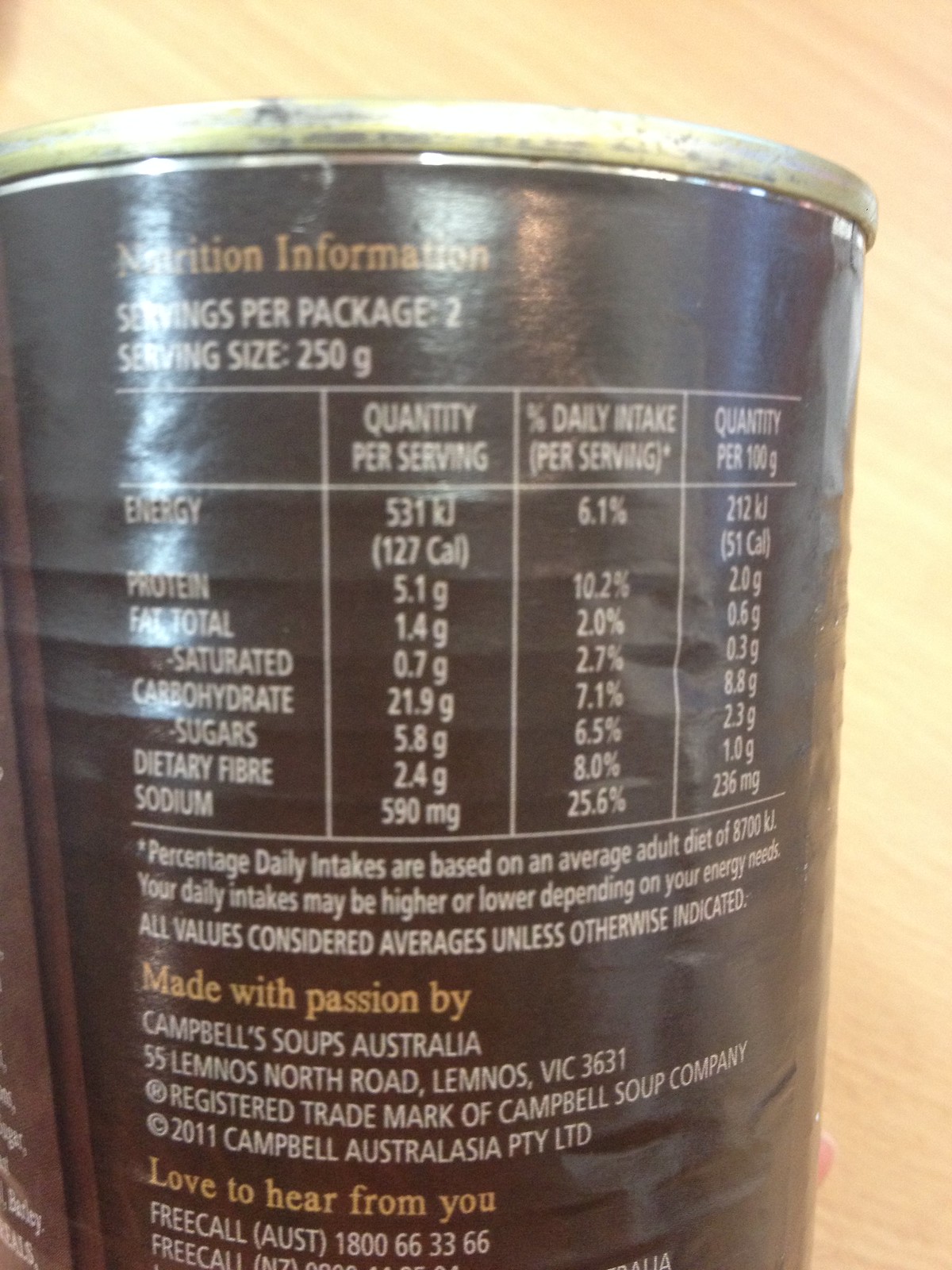The portrait-mode color photo features the back label of a can of food, set against a light brown background that appears to be wood paneling. The can’s label is predominantly black, accentuated by a visible silver rim at the top. At the top of the black label, the heading "Nutrition Information" is written in brown, followed by white text detailing "Servings Per Package: 2" and "Serving Size: 250 grams." Below these details, there is a standard nutritional chart suggesting that the contents are a type of soup. Toward the bottom of the label, an orange inscription reads "Made with Passion by," followed by "Campbell's Soups, Australia" in white text.